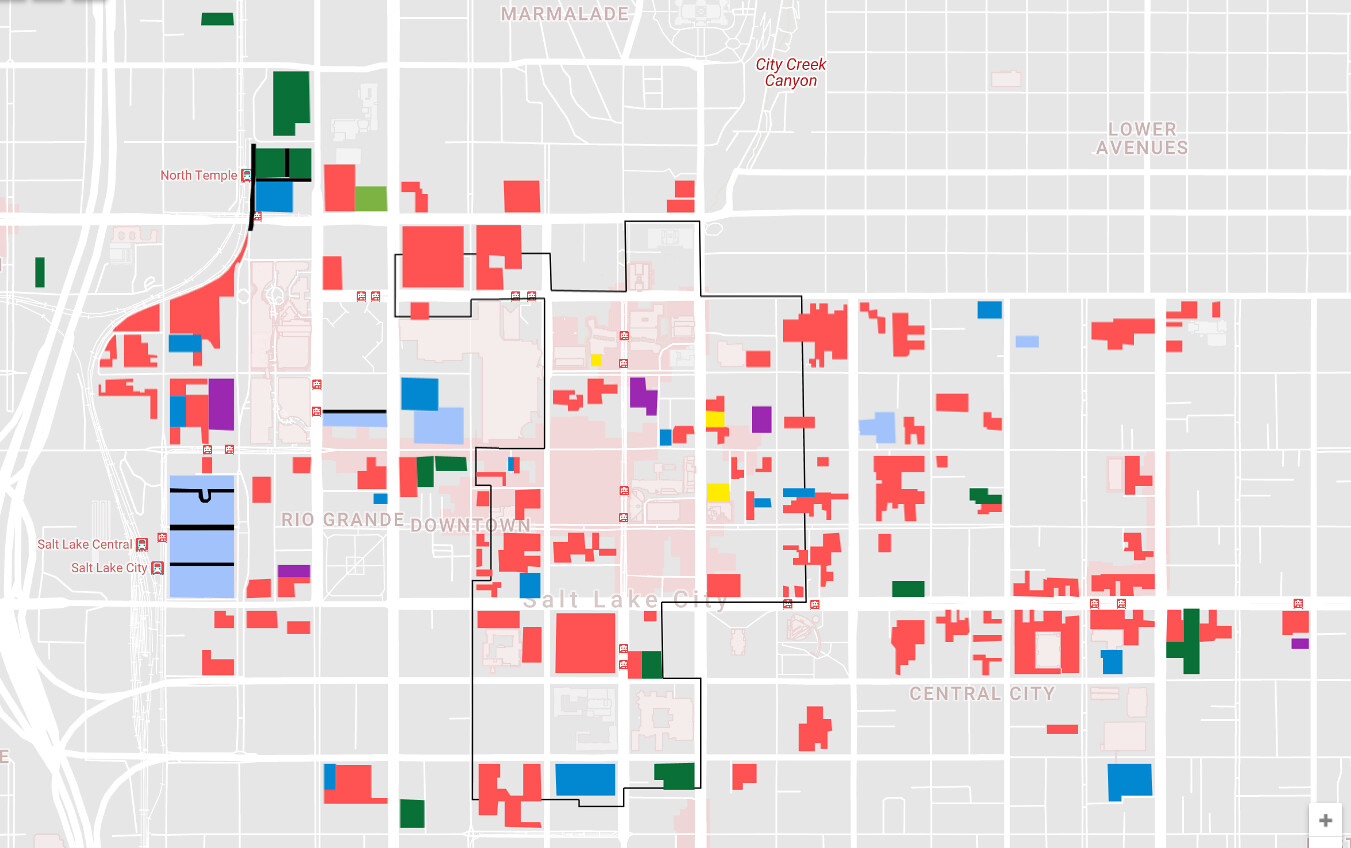This image appears to be a detailed town map, characterized by its use of various colors and shapes to denote different areas and elements. 

On the right side, larger rectangles are delineated by white lines, filled with a mix of white, blue, and variously colored blocks—ranging from red and purple to green and shades of blue. 

The central part of the image focuses on a floor plan composed primarily of blue squares and rectangles, interspersed with some red and pink blocks. Notably, there's a distinctive shape in the center, resembling two connected triangles, surrounded by numerous pink-shaded blocks with additional red and blue blocks towards the bottom.

Towards the top of the image, a variety of smaller blocks in colors like red, blue, and pink are evident. Meanwhile, the left side features an assortment of squares and rectangles, with the upper smaller squares containing no designs, instead labeled with terms like "AdWords," "OA," "OFA," and "menus." At the bottom of this section, larger rectangles also display a mix of blue, red, and green colors.

Overall, the map incorporates a diverse palette and geometric patterns to represent various town elements, possibly indicating different buildings, sections, or features within the town.